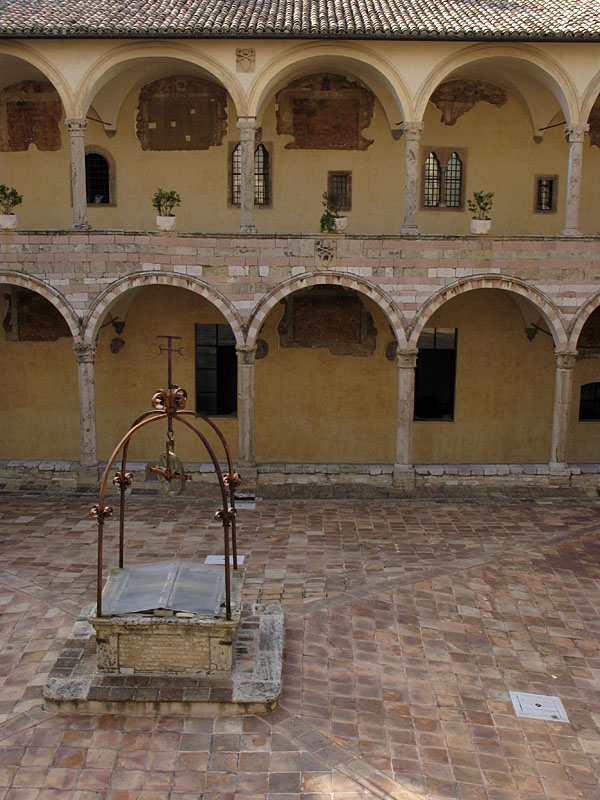The photograph captures an outdoor courtyard, presumably the interior space of a possibly abandoned building. The ground is paved with brown stone tiles arranged in a square pattern, and there appears to be a slight upward incline towards the center. At the heart of the courtyard stands a covered well, made from small white bricks, topped with large double metal doors and an overhead metal rod with a pulley mechanism, suggesting its past use as a functional well. The building's yellow-beige walls frame the courtyard, featuring multiple multi-pane windows, some of which appear boarded up, adding to the sense of abandonment. The structure spans two stories, with arched columns visible on both levels and a tiled roof capping the top. The walls exhibit signs of wear with fading and cracking paint, enhancing the aged and neglected ambiance of the scene.